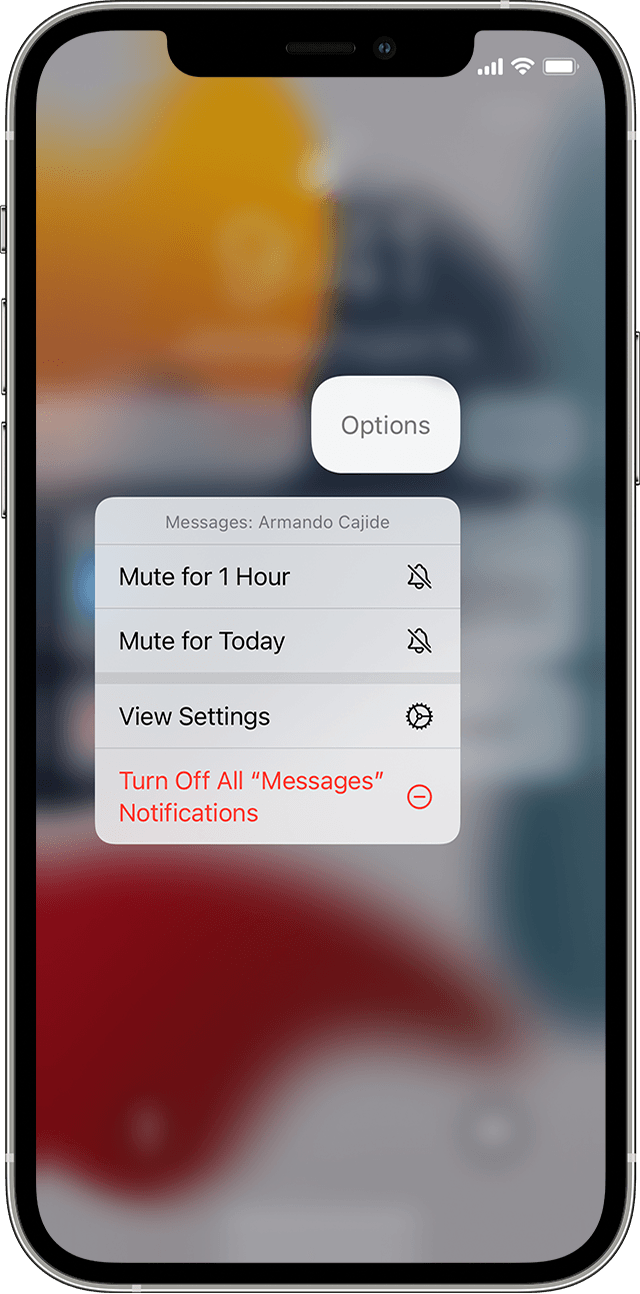The image showcases a complete cell phone, revealing both the physical device and its screen. The background image on the screen is blurred but composed of various colors, adding an abstract aesthetic. Prominently centered on the display is a pop-up menu. Directly above this menu, a button labeled "Options" is visible.

Occupying roughly one-quarter of the screen from top to bottom and extending two-thirds across the screen from left to right, the menu features a gray background. At the top of the menu is the text "Messages, Armando, LAD," followed by several selectable options. The first option is "Mute for one hour," directly below which is "Mute for today." These options are separated by a thin gray bar, adding visual separation and clarity. Below this separator is another option labeled "View Settings." At the bottom of the menu, a final choice reads "Turn Off All Messages Notification." 

All these menu options are superimposed over the blurred background, indicating an active state with the possibility to select and interact with any of the available options.